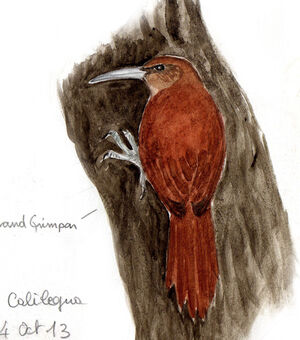The painting depicts a striking woodpecker perched on the side of a brown tree trunk, set against a simple white background. The trunk, depicted at an upward angle to the left, features meticulously shaded bark in various hues of brown, suggesting a textured surface. The woodpecker, rendered in vibrant red with rust-colored and light brown tones, stands out against the tree. Its head is predominantly red, with a hint of black around the eye, and a light brown or tan breast. The bird's beak is a grayish-white with a touch of red on the tip, while its large, white claws grip the tree bark firmly. The artist's skillful use of shading brings out the detailed feathers and lines of the bird. In the lower left corner of the image, the number 13 is visible, along with a partially cut-off word "I-M-P-A-N" and the signature "Regina," possibly indicating the artist. The painting's two-dimensional quality captures the essence of the bird and tree in a flat but vividly detailed manner.